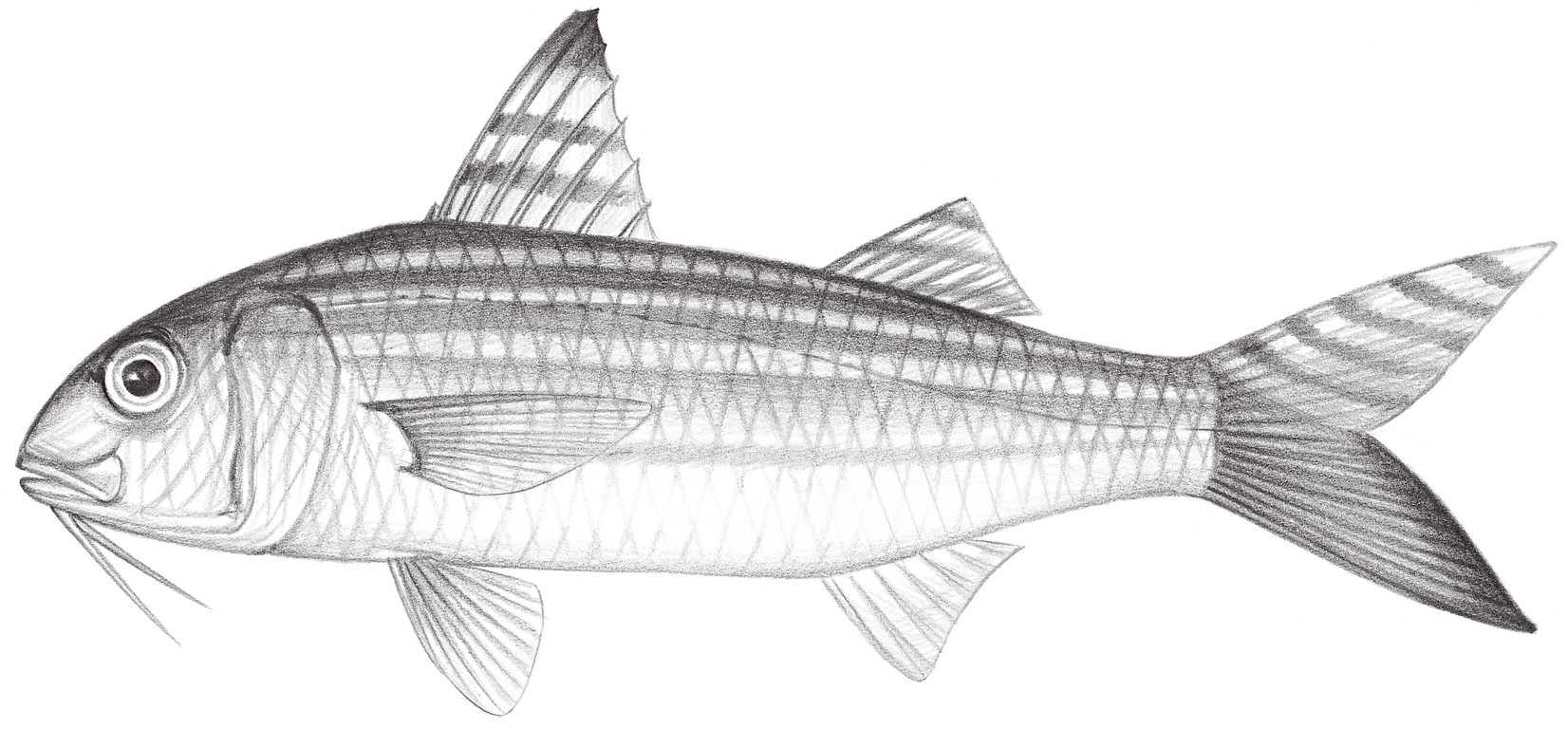The image depicts a highly detailed, hand-drawn, pencil sketch of a large fish, centered against a completely white background, with no text present. The fish, oriented with its head to the left and its tail to the right, displays intricate black, white, and gray shading. The scales of the fish reveal a detailed crisscross or checked pattern, giving it texture and depth. The fish features multiple fins, including a prominent dorsal fin on the top, additional fins on the bottom and side, and noticeable whiskers protruding from below its mouth. Its large, black, beady eye is open and encircled by rings, contributing to the lifelike appearance. Horizontal striping and consistent patterning extend to its tail, further enriching the visual interest of the drawing. The artistic style is illustrative, making it similar to depictions found in manuals or textbooks. This portrayal suggests it could be the work of a professional artist or an adept amateur, suitable for display in settings such as homes or sporting goods stores.